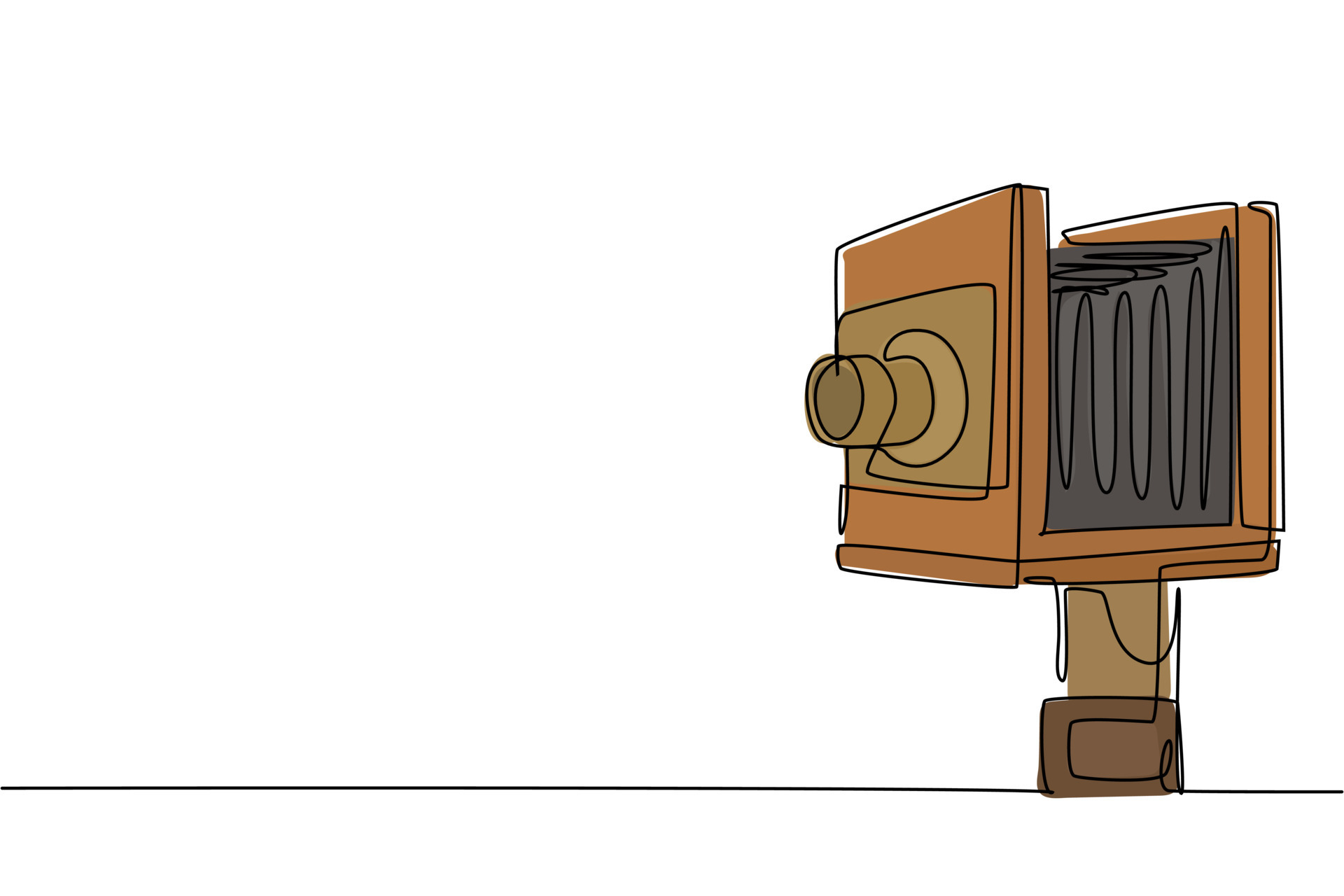This is a simple illustration designed to resemble an antique camera icon, possibly for use as an asset on websites or videos. The image features a collapsible antique camera predominantly situated on the right side, facing left, against a stark white background. 

The camera is characterized by its black fabric bellows with an accordion-like appearance at its center and a singular lens protruding from a square front element. The body of the camera is depicted in varying shades of brown to mimic a wooden texture, with the top part of the camera open, revealing folded dark gray material within. 

Despite its simplicity, the illustration uses basic shapes and lines to represent the camera's structure effectively. A solid horizontal black line runs across the bottom of the image, grounding the composition. Overall, the drawing employs unembellished colors and clean lines to clearly convey the antique camera's distinct features.